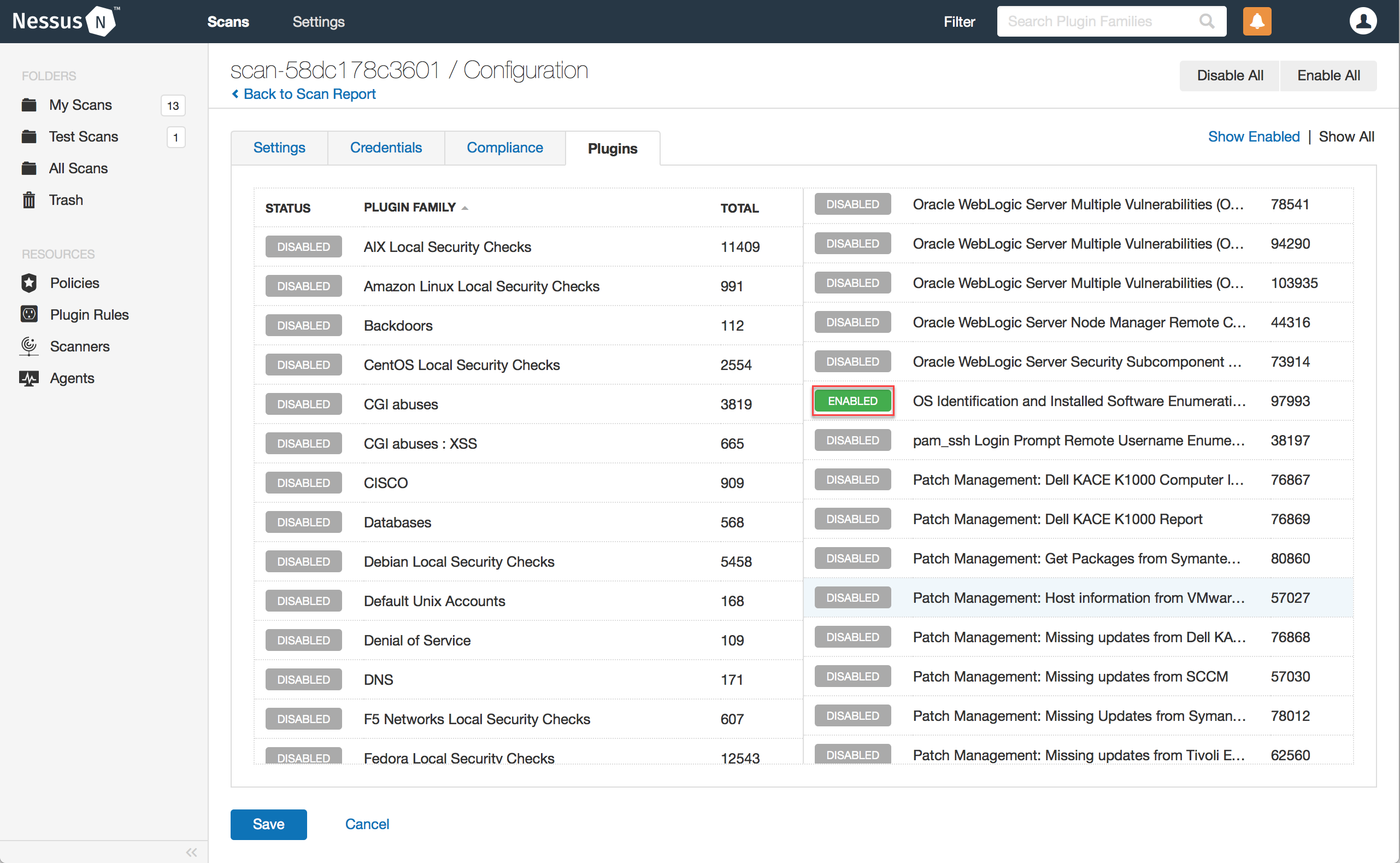The image depicts the Nessus security platform interface. At the top of the screen, a black banner prominently displays the Nessus logo, consisting of a white hexagon with a capital "N" inside. The banner also includes navigational elements labeled "Scans" and "Settings" in white text. On the right side, there are a filter option and a search bar labeled "Search plug-in families," accompanied by a magnifying glass icon. Additionally, notification icons such as a bell, a square, and a circle with a person icon are present.

On the left side of the interface, the navigation panel includes options like "My Scans," "Test Scans," "All Scans," and "Trash." Above these, in gray text, it says "Folders," and below, it lists "Resources," "Policies," "Plugin Rules," "Scanners," and "Agents," all in black text. Notably, there are 13 "My Scans" and 1 "My Test Scans."

The main workspace on the right features a white background detailing a specific scan identified as "scan-58DC178C3601/configuration." A link titled "Back to Scan Report" is displayed in blue. Below this, there are tabs for "Settings," "Credentials," "Compliance," and "Plugins," with the "Plugins" tab currently active. At the top of this section, headers read "Status," "Plugin Family," "Total," and "Status." The table below these headers contains numerous entries, corresponding to various plugins and configurations.